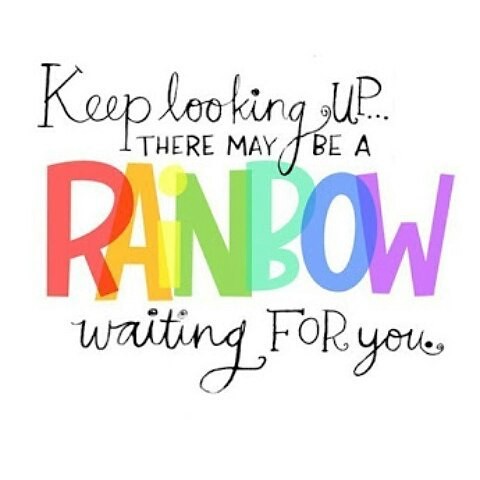This is a simple and vibrant graphic image on a white background. At the top, in black handwritten script, it reads "keep looking up..." Below this, in smaller black handwritten text, it says "there may be a." Underneath, the word "rainbow" is written in bold, multicolored letters: R is red, A is orange, I is yellow, N is green, B is teal green, O is dark blue, and W is purple. The phrase concludes with "waiting for you" in black script at the bottom. The overall design has a charming and whimsical feel, typical of a cute poster or inspirational sign, with the colorful "rainbow" standing out prominently amidst the handwritten text.